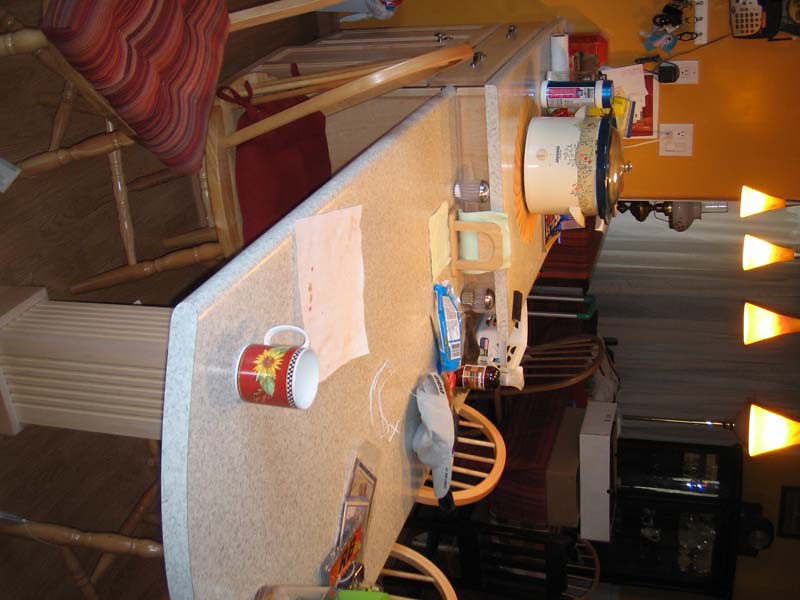The image depicts a modern kitchen scene where the focus is on a sleek, white marble countertop and an adjacent table. The image is rotated, making the countertop and table's edges face the right side of the horizontal frame. Centered on the countertop is a large white electric pot. The attached table, sharing the same white surface with subtle grey markings, seamlessly extends from the cabinetry below the countertop. 

On the left side of the table, two chairs with vibrant red cushions are slightly pulled away from the table. Positioned directly opposite, two wooden chairs are neatly aligned with their backs against the table's edge. 

Resting atop the countertop is a coffee cup and a bag of some food item. The tabletop hosts a collection of baseball cards and a set of keys, adding a personal touch to the scene.

Above, four light fixtures hang, casting a warm glow over the area. In the background, white curtains elegantly frame another wooden chair and a stacked pair of boxes. The entire scene is set against a backdrop of a rich brown wooden floor that extends underneath the table.